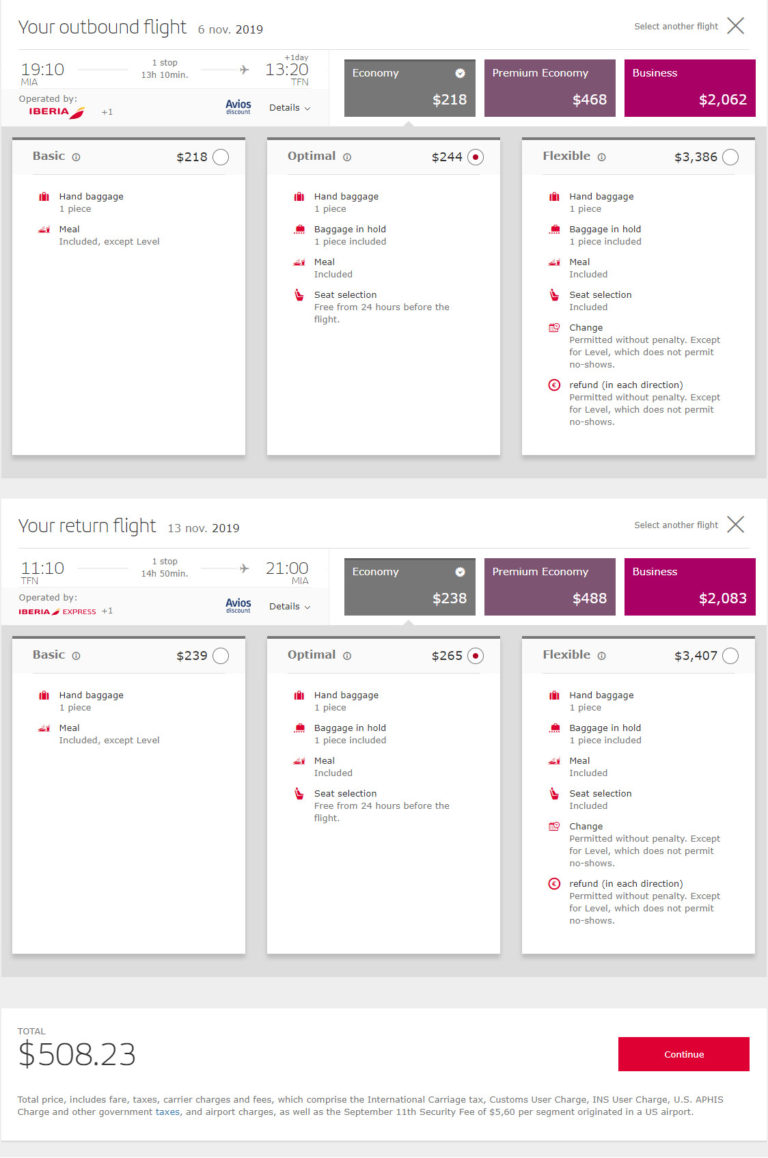The image depicts a screenshot from a flight booking website. At the top, the header "Your Outbound Flight" is clearly visible with a date of November 6, 2019. Below this banner, there are three color-coded options presented in boxes: a gray box for the "Basic Flight," a purple box for the "Optimal Flight," and a pink box for the "Flexible Flight." Each option has associated prices and clickable circles for selection. The costs are listed as $218 for the Basic Flight, $244 for the Optimal Flight, and a considerably higher $3,386 for the Flexible Flight.

Further down the page, "Your Return Flight" is shown with a date of November 13, 2019. This section mirrors the outbound flight layout, featuring the same three color-coded options with corresponding detailed descriptions and selection circles.

At the bottom, the total price for the selected flights is prominently displayed in bold black text: $508.23. To the right side of this total, there is a bright orange button designed for users to confirm and finalize their flight selections.